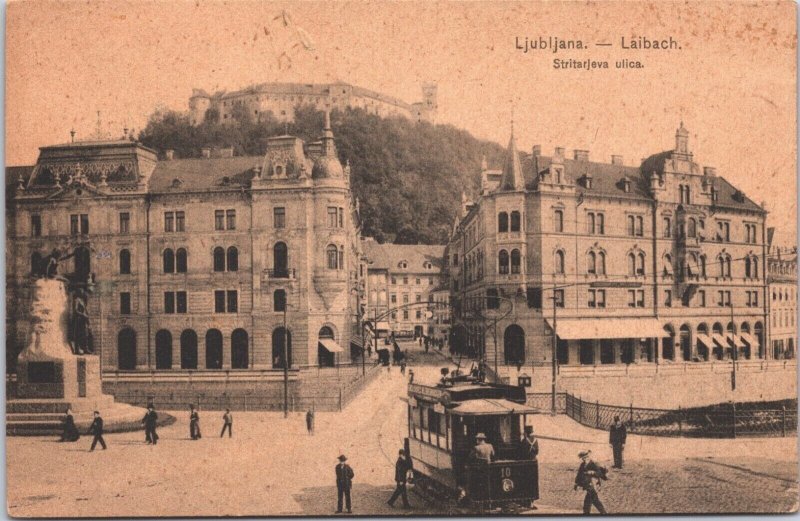This is a black-and-white photograph resembling a postcard, taken outdoors in an old city street. The image, heavily aged with an off-white or pinkish tint, prominently features two stately and ornate buildings flanking a bustling central thoroughfare. In the very top right corner of the photograph, black text reads "LJUBLJANA - LAIBACH," followed by "STRITARJEVA ULICA," indicating its location.

In the middle of the street, a trolley car heads towards the viewer, with a few men visible both aboard and around it, dressed in early 20th-century attire—long sleeves, hats, and business suits. On the left side of the image, a woman and four men walk along the sidewalk past a significant monument. This monument comprises two granite blocks and rises to about two stories, tapering towards the top where winged figures or statues might be discerned.

The building on the right is a four-story structure made of brick or stone, featuring a gabled roof, a spire, awnings, and first-floor arches, portraying a stately and grand architectural style. Across from it, the building on the left also boasts a spire and man side roofs, with similar arches on its first floor and three upper flights.

Between these buildings and further in the background is another four-story building with a gabled roof. In the far distance, atop a hill, a large structure akin to a castle or palatial estate looms, completing the timeless and grand ambiance captured in the photograph.